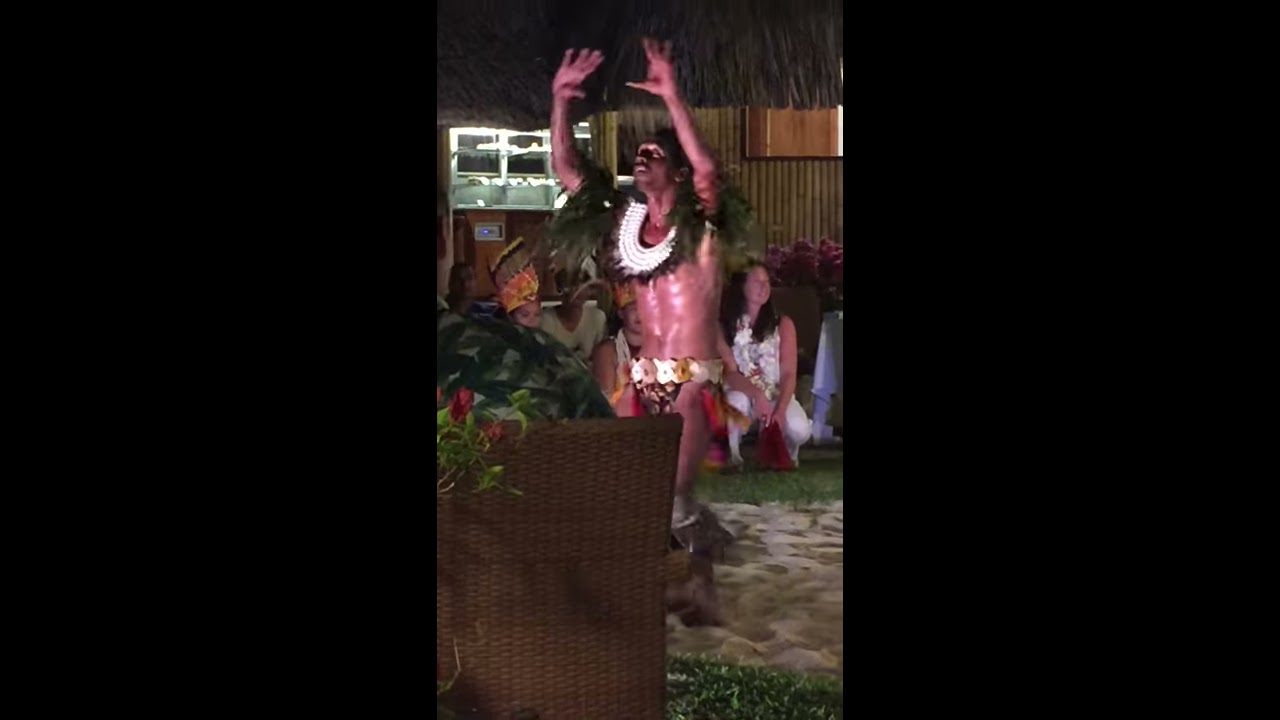The photo features a nighttime outdoor performance framed by blacked-out left and right thirds, creating a border around the central image. In the lower left corner, the back of a wicker chair is visible, occupied by a man whose shoulder is seen as he watches the scene. Central to the photo is a brown-skinned man, bare-chested, adorned with a striking white beaded necklace and grass-like coverings on his shoulders. He has a gold-colored metal belt around his waist, with a black cloth hanging down, and his feet are bare, encircled with similar grass coverings. The man is captured mid-dance, with his arms energetically raised and fingers splayed, looking upwards. He is dancing on sand, which appears to be part of a Hawaiian luau. Behind him, several women in traditional Hawaiian attire are seated, and the backdrop includes a bamboo-style hut with a grassy roof, reinforcing the Hawaiian theme.